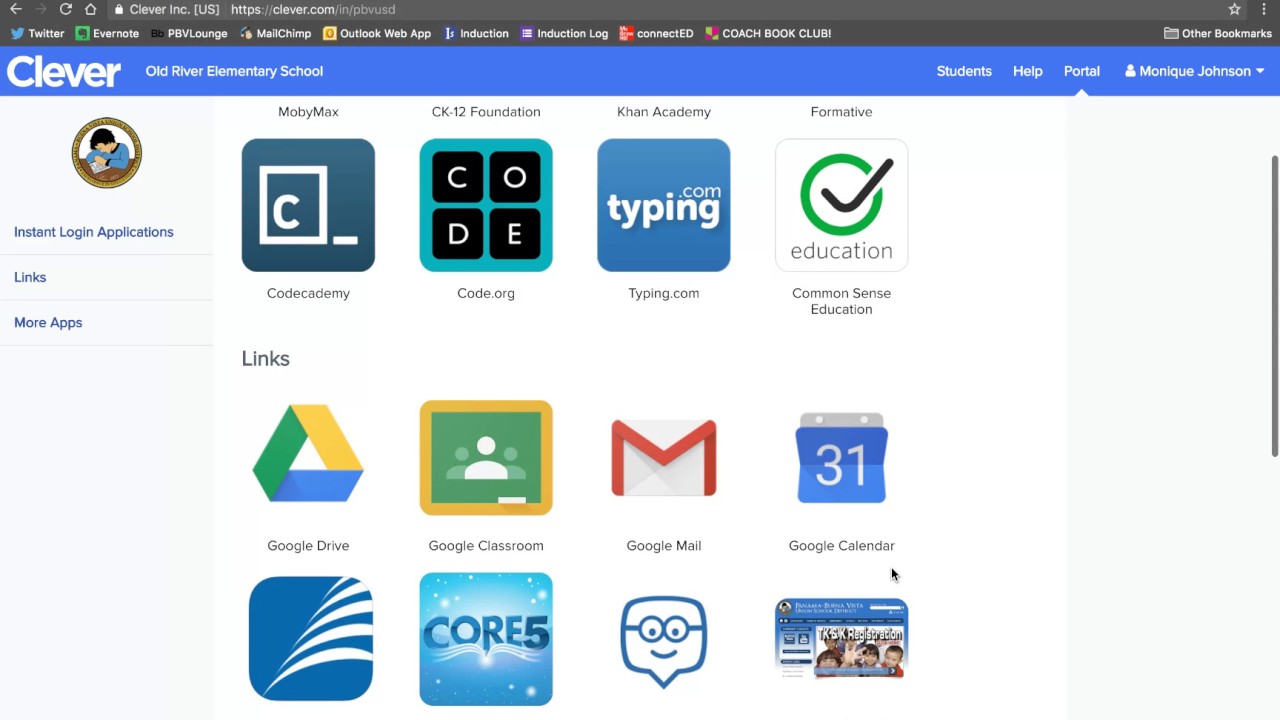This digital screenshot showcases the Clever portal for Old River Elementary School. Featured prominently is Monique Johnson’s user profile. The interface includes various educational application icons such as Code Academy, Code.org, Typing.com, Common Sense Education, and Education.com. Additionally, it provides access to Google Drive, Google Classroom, Google Mail, and Google Calendar, marked with the date "31." There is also a link to Core 5. The website URL displayed at the top of the screen is https://clever.com/in/pbvusd.